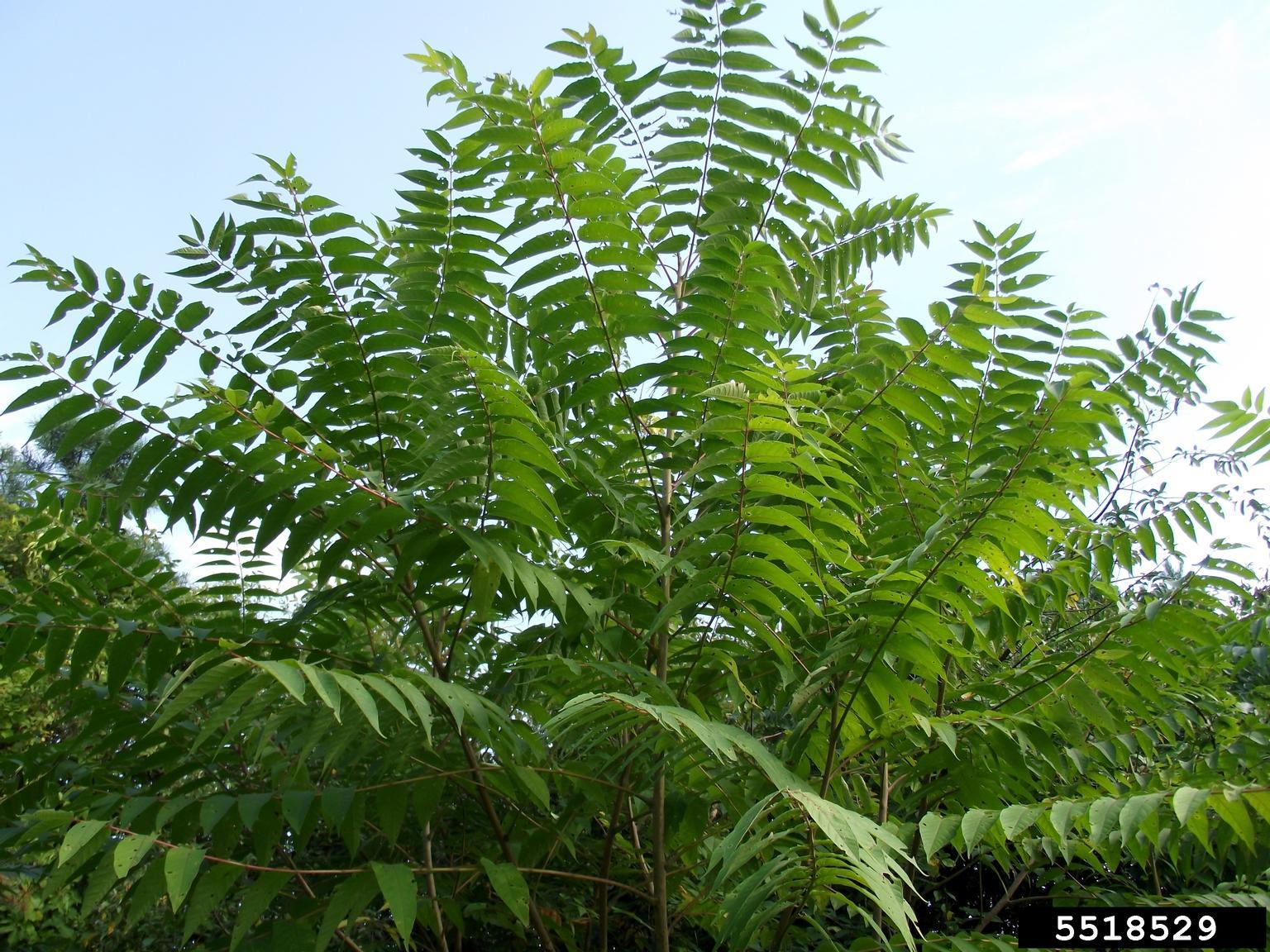In this detailed image, we are presented with a vibrant outdoor scene showcasing a large tropical plant or tree, prominently displayed from a front-facing viewpoint. The plant has an impressive array of stems and branches protruding in every direction, sporting lush green leaves that vary in shade from lighter to darker greens, hinting at a diversity of plant types or differing sunlight exposure. Amidst the foliage, some brown stems are visible, adding depth to the plant's structure. The setting appears to be a dense forest or jungle, as suggested by the numerous similar trees in the background, creating an immersive natural atmosphere. Clearly, this photograph was taken during the daytime, under a predominantly clear sky, with minor clouds observable on the right, contributing to the serene ambiance. Noteworthy details include the sequence of numbers "5518529" in white text on a black background, discreetly positioned at the bottom right corner of the image.